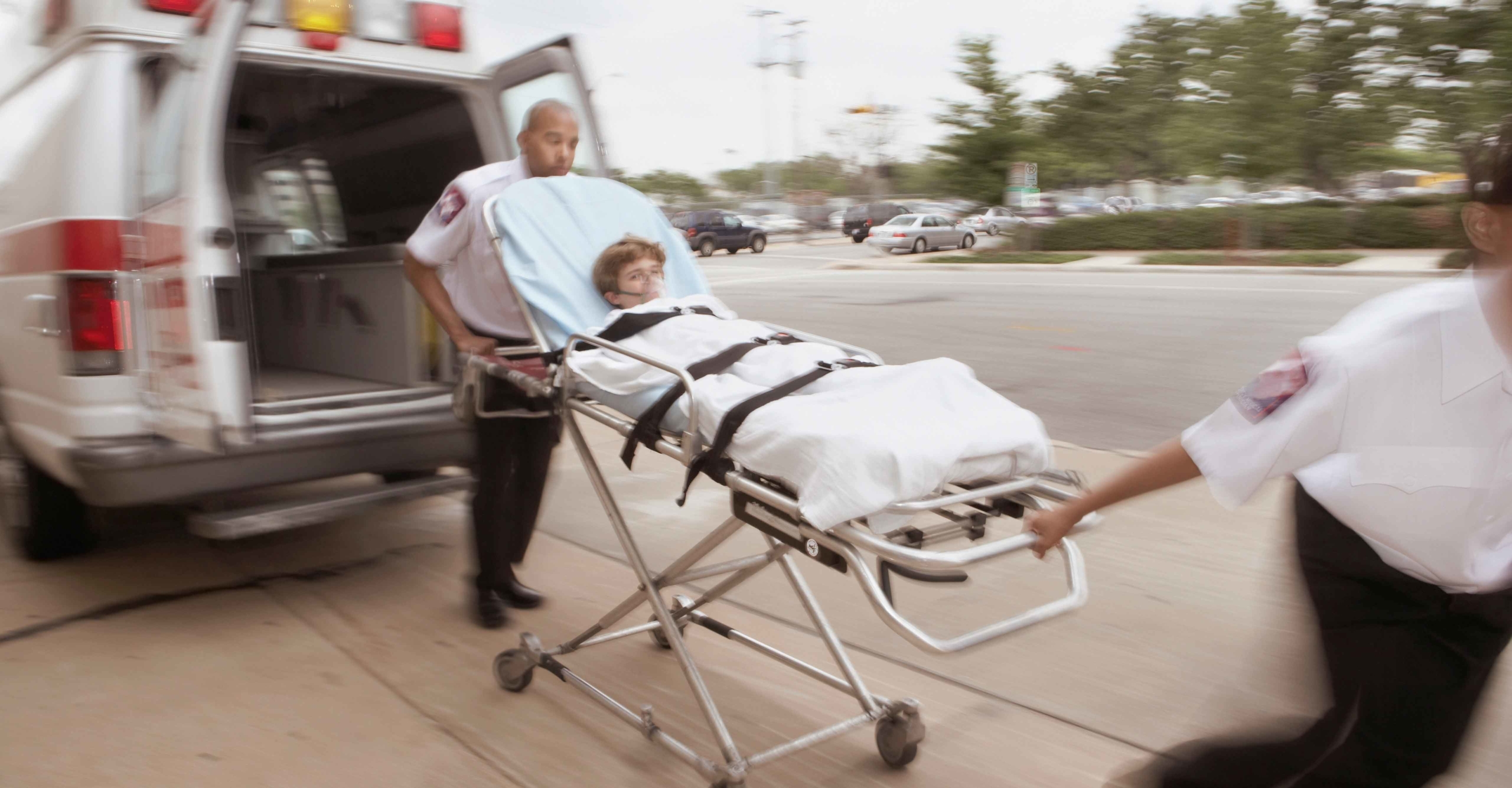In this landscape-oriented image, a young Caucasian boy, likely around ten years old with brown hair, is strapped to a stretcher covered in a white blanket. An oxygen mask covers his mouth, and he is secured with three seat belts. The scene captures two EMT personnel, one at each end of the stretcher, maneuvering him towards the back of an open ambulance. The EMT at the head of the stretcher, a black man wearing black pants and a white shirt with an insignia on his sleeve, is pushing from behind, while the one at the foot, a woman in similar attire, pulls from the front. The background reveals a blurred mix of sidewalk, trees, street, cars, and sky, indicating a sense of urgency and movement as they prepare to transport the boy to a medical facility.